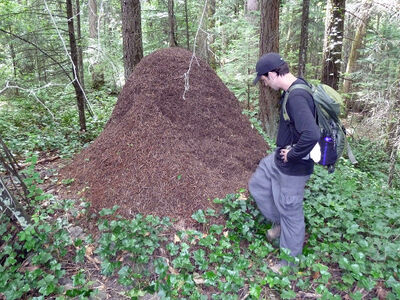In this photograph, a man is exploring a dense forest, where he encounters an imposing, brown dirt mound that stands slightly taller than him. The man, dressed in a dark blue long-sleeved shirt, light gray cargo athletic pants, and a dark cap, gazes intently at the mound, which has a noticeable hole about midway up, possibly indicating it as an animal's burrow. He carries a dark backpack, with a water bottle visible, and might be holding a canteen in his hand. The setting is rich with green vines sprawling across the forest floor, and numerous tree trunks fill the background. Some trees are bare, with empty twigs and branches hanging lifelessly. The overall atmosphere suggests a calm, overcast day in the heart of the forest.